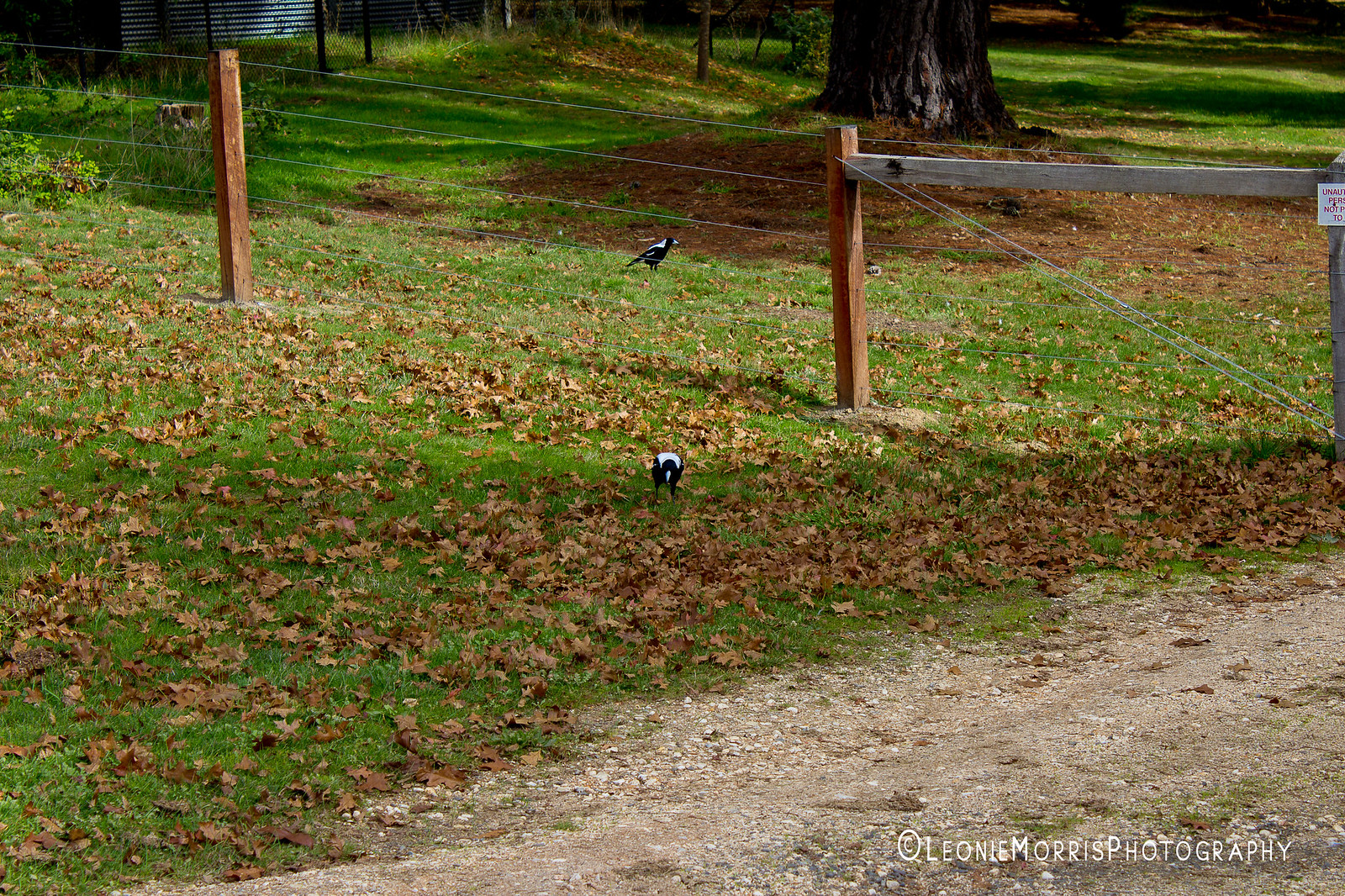This image captures a serene outdoor scene, possibly in a farm or park reserve setting, dominated by a green grassy field interspersed with fallen brown leaves. Running horizontally across the image is a fence with evenly spaced wooden posts connected by six thin metal wires. A prominent large tree stands majestically near the top of the image, adding to the natural ambiance. A dirt path with scattered rocks stretches diagonally from the lower right corner almost to the left edge of the image. There is a small sign on one of the posts that might indicate a gate, featuring distinct vertical or diagonal wires. In the background to the left, there is a glimpse of a building adding depth to the scene. Two black and white birds are centrally positioned, one on each side of the fence, enhancing the pastoral charm. The photograph is credited to Leonie Morris Photography, marked clearly in white text along with a copyright symbol in the bottom right corner. The setting suggests it is mid-day, with ample natural light illuminating the scene.